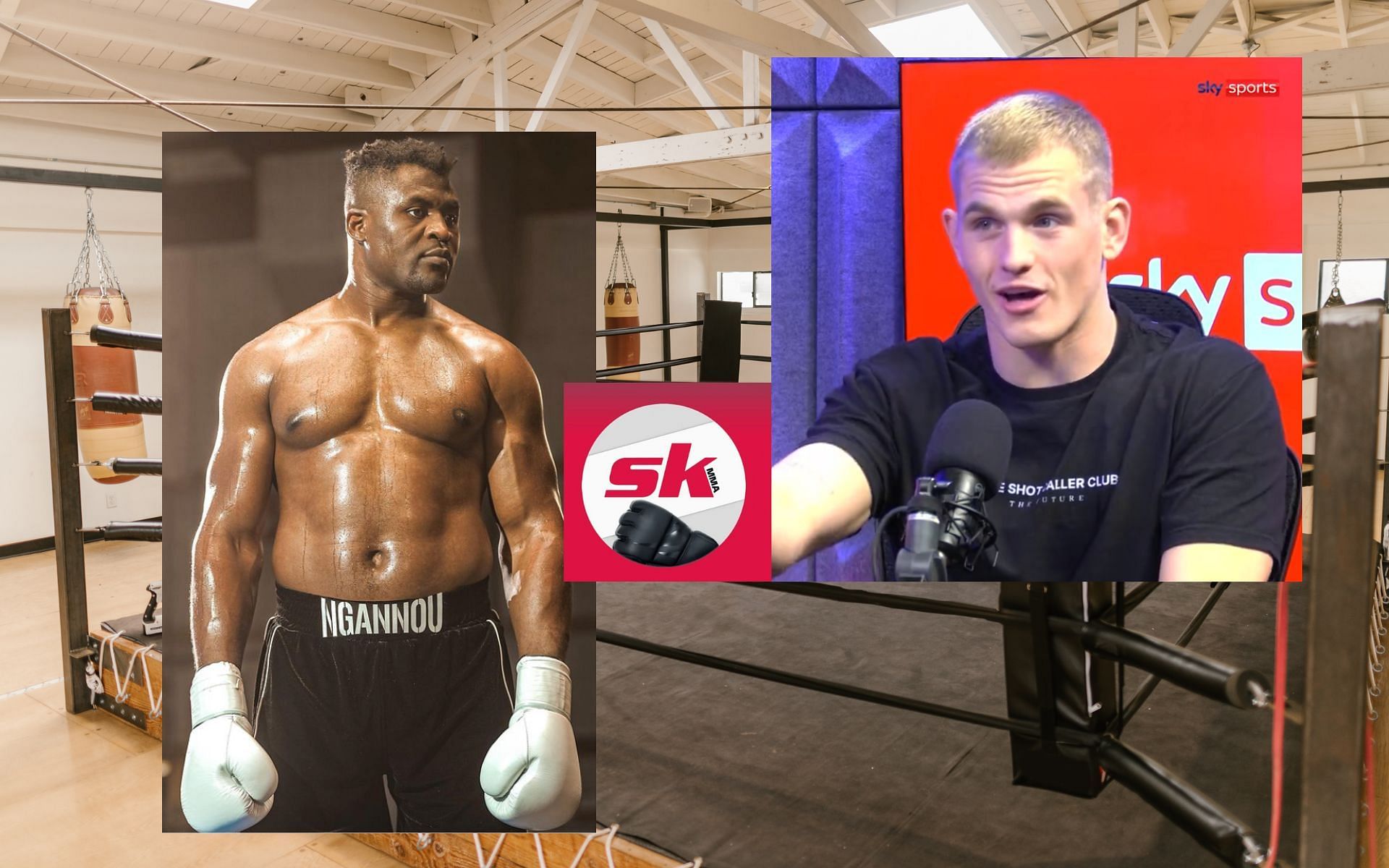The split image features two distinct sections. On the left, a striking photograph captures a black boxer, exuding strength and focus. Possessing a well-defined muscular physique, he is adorned with white boxing gloves and his skin gleams with oil. His short, cropped hairstyle, longer at the top, complements his intense expression as he gazes sideways, highlighting his chiseled form. The backdrop is an abstract composition of brown hues, with various shades of tan subtly blended in. Superimposed over this image is a scene of a boxing gym, characterized by its sprawling brown floor and high, unfinished vaulted ceilings where exposed beams, lights, and sporadically hanging boxing bags are visible.

On the right, another figure appears—a white man, possibly another boxer or an announcer. He stands before a large microphone, speaking with a certain authority. A distinctive red box bearing the letters "SK" in a white circle and a black object that appears to be a microphone, is positioned next to him. His background features a vertical purple stripe on the left against a predominantly red backdrop. This man has blonde hair, adding a contrasting element to the visual narrative of the image.